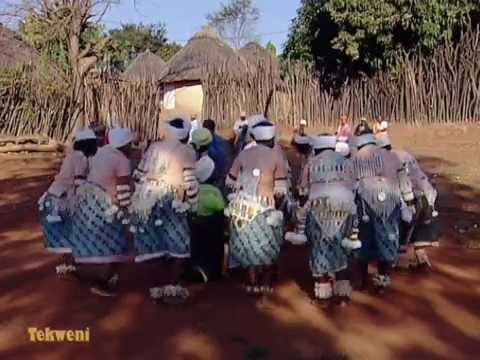The image captures a group of black women standing in a huddle, possibly in Africa, in front of thatch-roofed huts scattered across a reddish-brown dirt ground. All the women, whose faces are not visible, are dressed in culturally distinctive attire: white headscarves, beige-to-pink tops, and blue skirts adorned with black markings and white ornamentation. Some white shawl-like items are tied around their waists, and fuzzy, beaded anklets wrap around their bare feet. They appear to be looking toward a centralized point, possibly indicating an activity or dance. The scenery includes sparse trees and a clear blue sky in the background. The text "Tekweni" is prominently displayed in yellow at the bottom left corner of the image.